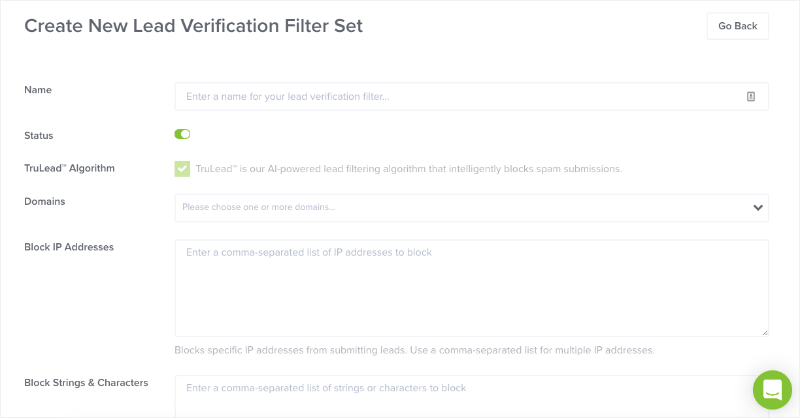Screenshot Description: Creating a New Lead Verification Filter

This screenshot depicts the interface for creating a new lead verification filter, likely part of a lead management or CRM system. The page is titled "Create New Lead Verification Filter Set," and features several interactive elements and fields, as described below:

1. **Navigation and Action Buttons**:
   - A "Go Back" button is prominently displayed, allowing users to return to the previous page if needed.

2. **Filter Naming**:
   - A field labeled "Name" with an instruction to "Enter a name for your lead verification filter," inviting users to specify a unique identifier for the new filter.

3. **Status Toggle**:
   - A toggle switch for the filter's status which can be set to either "On" or "Off." The current status is "On," indicated by the label "True."

4. **True Lead Algorithm**:
   - The option "True Lead Algorithm" is selected. A description beneath this option explains that "True Lead is our AI-powered lead filtering algorithm that intelligently blocks spam submissions."

5. **Domain Selection**:
   - A section titled "Domains" with a prompt to "Please choose one or more domains," allowing users to specify which domains the filter will apply to.

6. **IP Address Blocking**:
   - An input field for "Block IP Addresses," where users can "Enter a comma-separated list of IP addresses to block." This field is designed to prevent specific IP addresses from submitting leads.

7. **String and Character Blocking**:
   - Another input area for "Block Strings and Characters," prompting users to "Enter a comma-separated list of strings or characters to block." This is used to filter out unwanted submissions containing specific text patterns.

8. **Help and Support**:
   - In the bottom-right corner, there is a chat icon, likely representing a help or support feature where users can get assistance with setting up their lead verification filters.

Overall, this interface is designed to help users create and customize lead verification filters efficiently, ensuring high-quality and relevant lead generation by blocking spam and unwanted submissions.